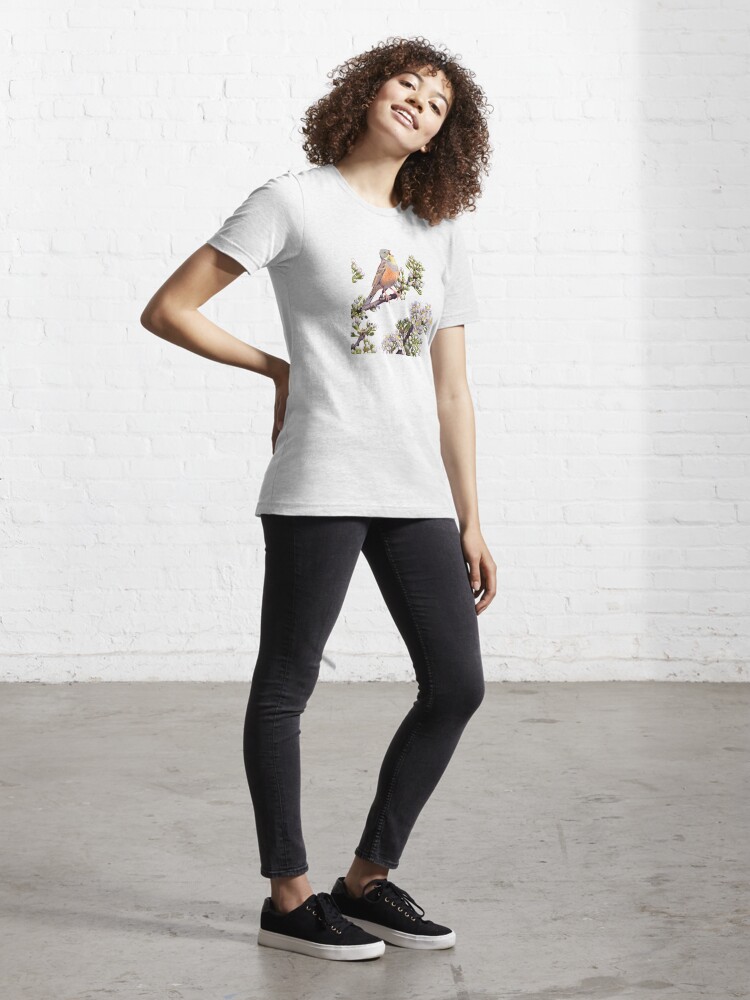The image captures a young woman in her mid-twenties standing comfortably in a vacant room with white brick walls and a gray concrete floor. She has a light complexion and appears to be of mixed African-American heritage. Her naturally curly shoulder-length hair is a golden dark brown. She wears light makeup and is smiling warmly, with her head tilted back slightly and cocked to her left shoulder. Her right hand rests on her hip, creating a bend in her arm, while her left arm hangs relaxed by her side. She stands with her left knee slightly bent forward and her right leg straight. Her outfit consists of a white t-shirt featuring an artistic bird with an orange chest perched on a branch with some green leaves, centrally placed on her chest. She pairs this with tight black pants or jeans and black sneakers with white soles. The scene is brightly lit, either by natural daylight or abundant artificial lighting, casting a shadow from her right foot, emphasizing the simplicity and tranquility of the setting.